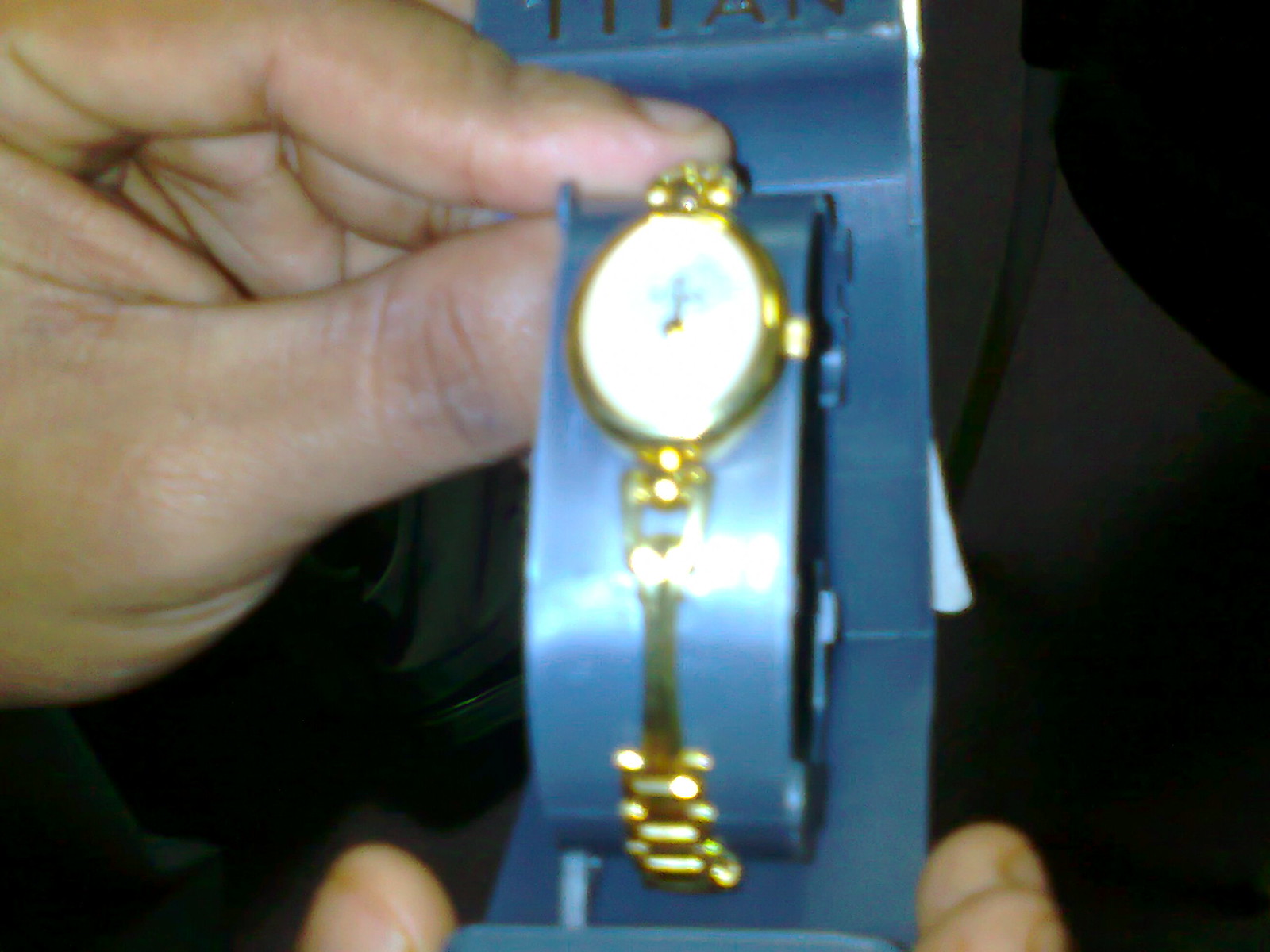The image depicts a close-up, albeit slightly blurry, of a gold woman's watch being presented in a blue (or bluish-gray) plastic display case. The watch, which exudes a delicate and ornate design with a thin chain-link band and a small, semi-oval shaped white face, is held by a man's hands. His left hand pinches the top of the case, with the thumb and forefinger visible, while his right hand cups the bottom. The watch features dainty black hands, including a winding mechanism on its left side, and rests on a protruding bump inside the case. The background is predominantly black, adding contrast to the scene, though details like a cut-off brand logo and a suggestion of a dirty floor in the periphery are vaguely visible due to the photo’s blurriness.